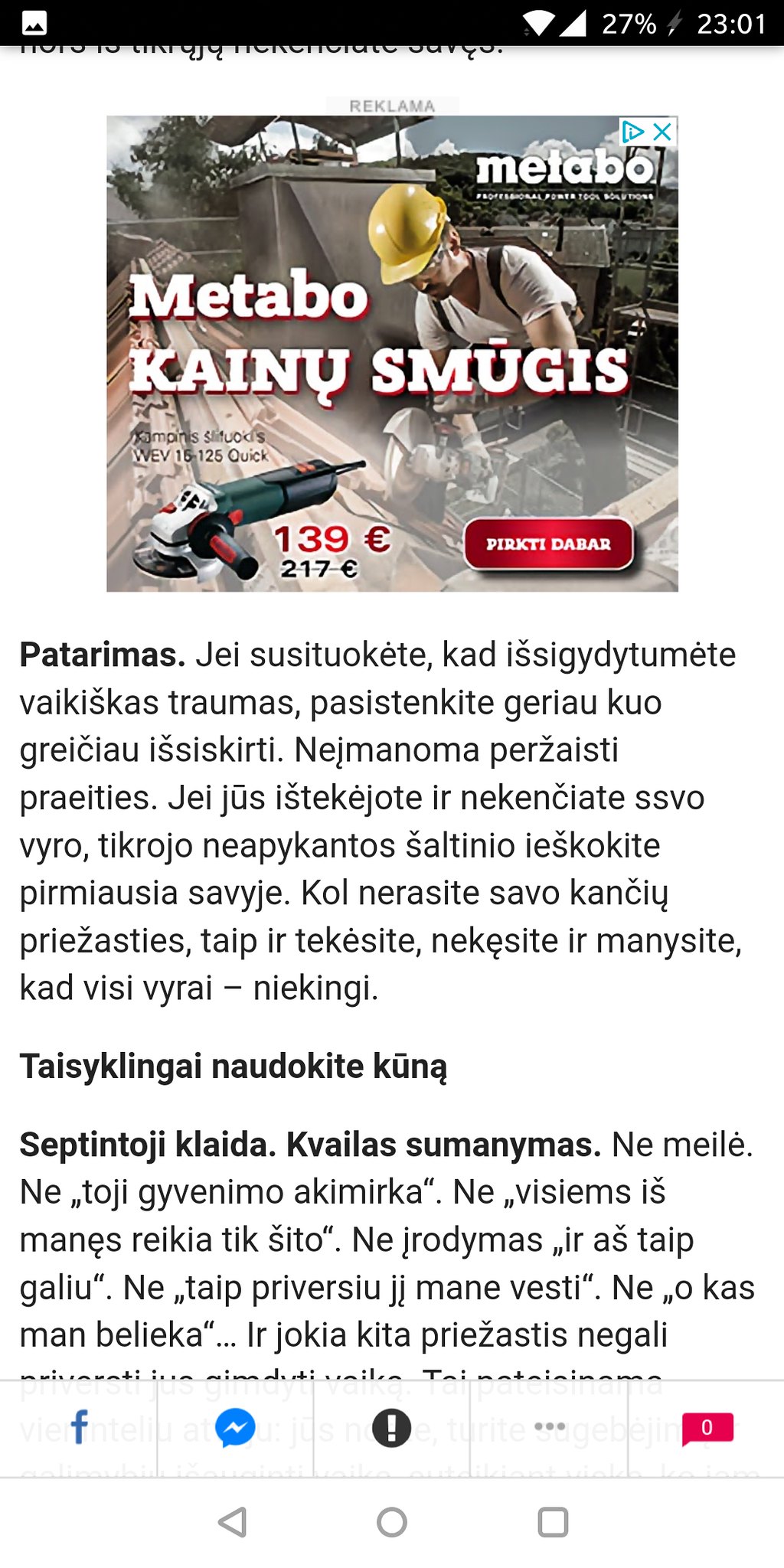The image is a detailed screenshot of a smartphone display showing a combination of a webpage or social media post, overlaid with an advertisement. At the top of the screenshot, the phone's status bar is visible, featuring a black bar on the left, an unspecified icon, a Wi-Fi symbol, a battery indicator showing 27% charge, and the time set to 23:01. Below this is the main content—an advertisement prominently positioned within a webpage or social media post.

The advertisement seems to showcase a construction worker actively engaged in his task, wearing a yellow hard hat and goggles. He is cutting wood with a saw, amidst a backdrop that includes a large metal dumpster and surrounding greenery. The ad text is in a foreign language, stating "Metabo Kenu Smugus" with the price listed at 139 euros, reduced from 217 euros. The ad also features a call-to-action button labeled "perktydarab."

Following the advertisement, the page contains additional content, including a couple of paragraphs written in the same foreign language. The paragraphs are interspersed with various symbols and text. At the bottom of the screenshot, more interface elements such as Facebook and Messenger icons are displayed, typical for sharing or interacting with the post.